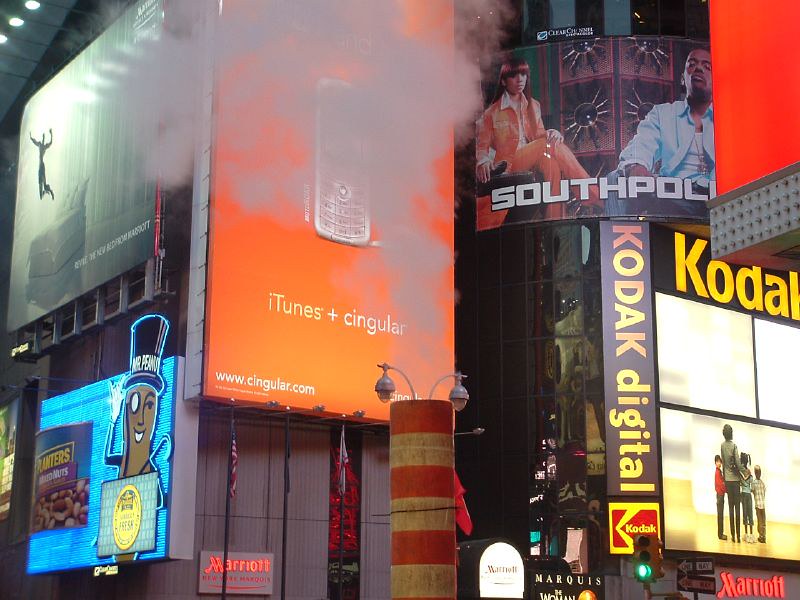This vibrant street corner scene captures a bustling urban environment teeming with advertising. Central to the image is a column of billowing steam emerging from a sewer grate, partially obscuring several signs. On the left, an imposing advertisement for the Marriott Hotel features an artistically rendered figure of a man jumping on a bed within a sleek, white hotel room. The Marriott logo is prominently displayed on the lower part of the building facade.

Adjacent to the hotel ad is an eye-catching three-dimensional billboard for Planters Peanuts. It showcases a curved peanut can filled with assorted nuts against a light blue backdrop, with Mr. Peanut himself, embossed and outlined in neon, extending from the can.

Dominating the middle section is a vertical billboard promoting iTunes and Singulair, featuring a sleek silver cell phone and the website "www.singulair.com" at the bottom. However, steam obstructs much of this detail. Nearby, a graceful glass structure suggests an atrium or garden foyer.

On the right, another striking advert pops out—a curved sign for the South Pole clothing brand. This ad features two stylishly dressed African American models: a seated woman in an orange suit and an orange jean jacket with orange pants, and a man in a light blue Oxford shirt layered over a white undershirt, accessorized with a necklace.

Further right stands a vertical Kodak Digital ad with the iconic Kodak logo, next to a more horizontal Kodak ad displaying a woman with three children, where one child looks at the camera while the woman looks away.

Foreground street details include a green-lit traffic light, a one-way street sign, and multiple American flags prominently positioned in front of the Marriott Hotel signage, adding a touch of patriotism to the urban chaos.